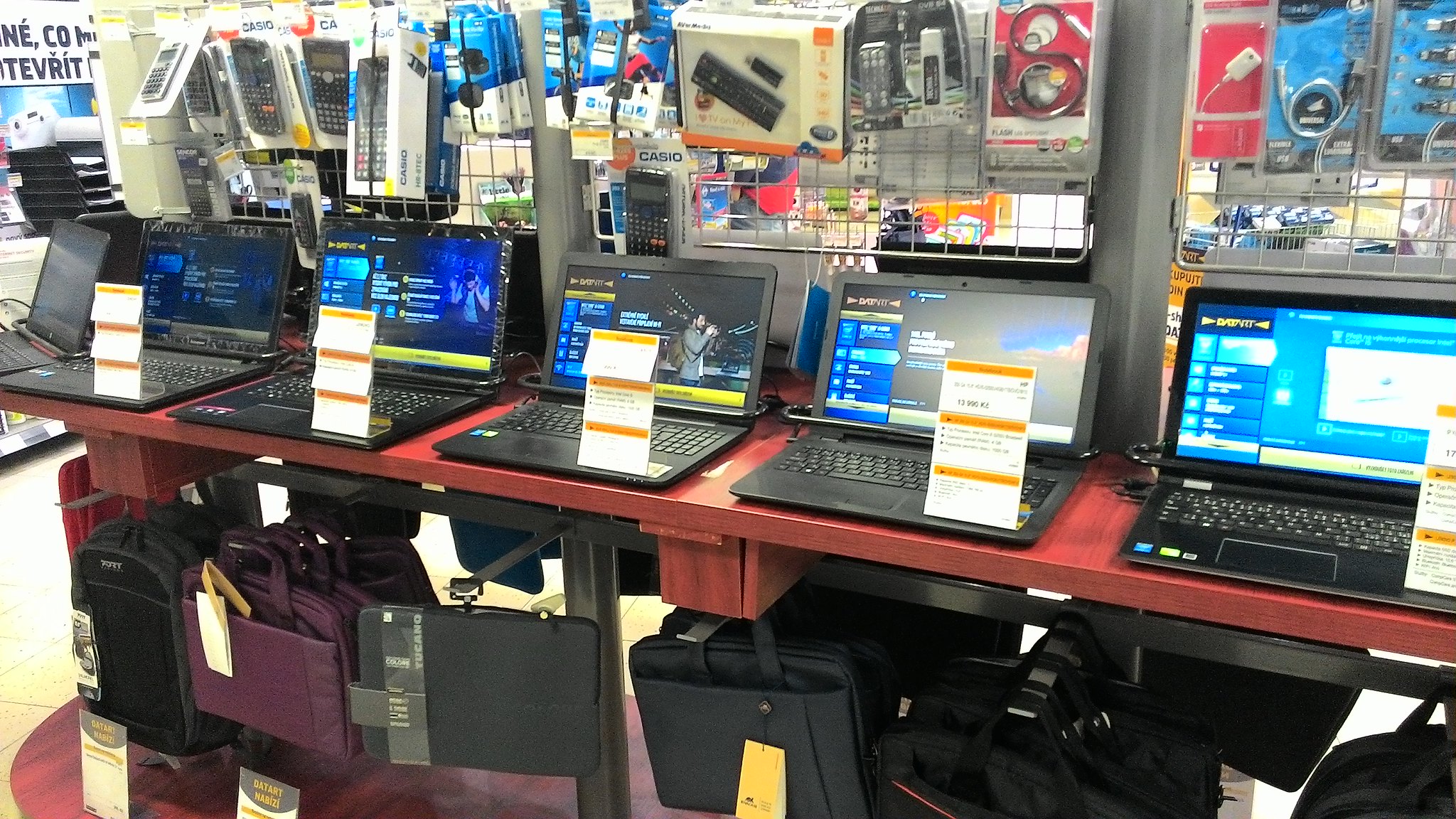In this real-life photograph of an electronics section in a retail store, six black laptops sit prominently on a wooden display table, all turned on with blue-themed screens. Each laptop has an informational card featuring a white background, black text, and an orange header, although the text is unreadable from the distance. Beneath the table are various laptop cases, primarily in shades of black, along with one in a distinctive plum color. Overhead racks above the laptops display an array of accessories, including HDMI cables, calculators, security cables, and keyboards. To the left, the photograph reveals a glimpse of the store's typical white tile floor and hints at another white and blue display with black writing in the background. The accessories on the rack are packaged in bubble wrap and cardboard boxes, offering a variety of small electronic products.